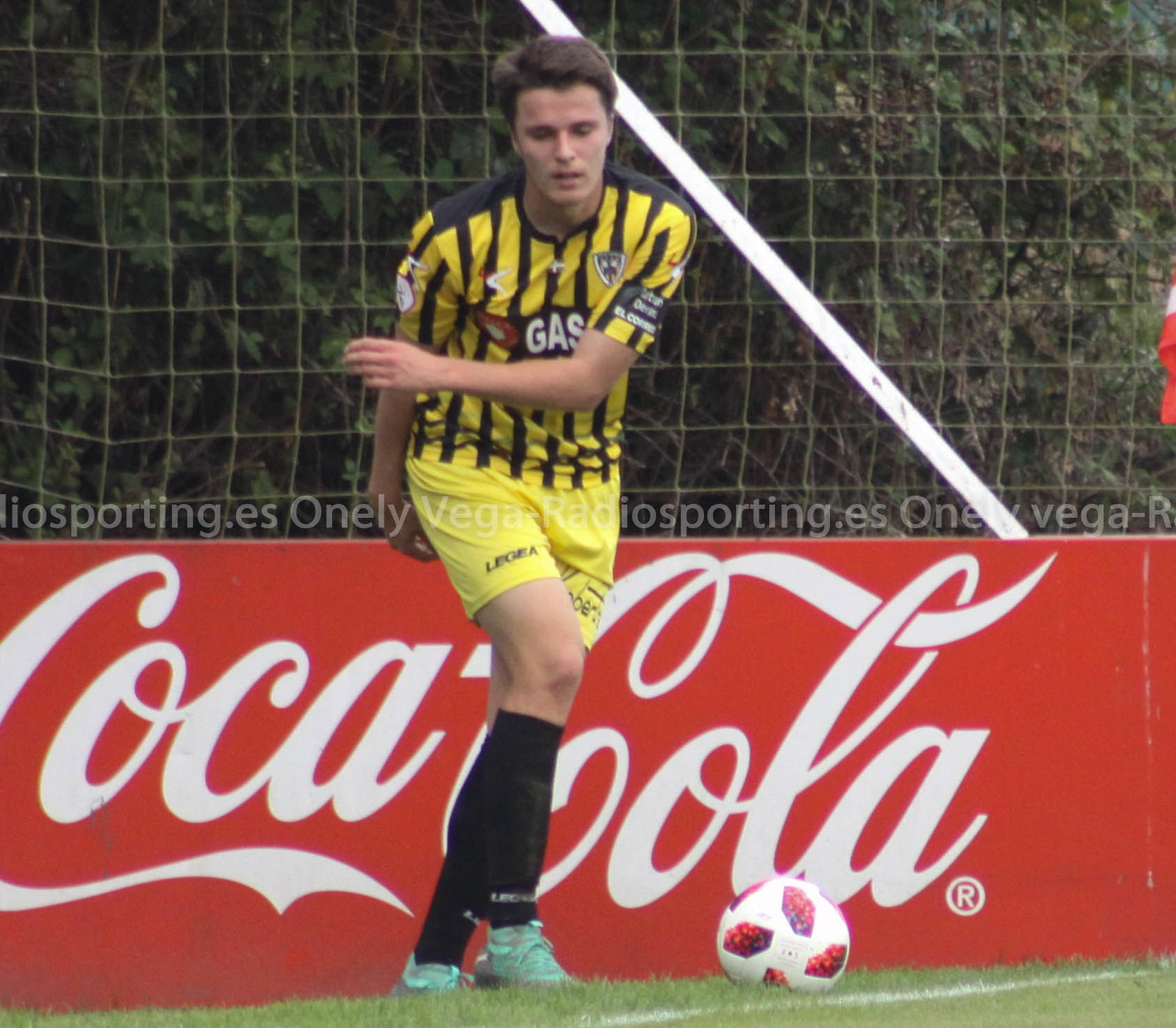The image captures a detailed scene of a soccer player poised to kick a ball on a sports field. The player is a young white male with slightly fluffy black hair, wearing a vertically striped yellow and black jersey marked with the word "Gas" on the center, matching yellow shorts, long black socks, and mint turquoise shoes. The soccer ball, which is white with red and pink panels, lies close to his right foot as he stands mid-stride, one arm folded to his side and the other extended back, ready to run and kick. In the backdrop, a red Coca-Cola advertisement in large white cursive letters stretches almost halfway up the image, sitting above a strip of green turf with a white line. Above this, a yellow net partially conceals a dense, dark green forest, adding depth to the scene. An angled white crossbeam is also visible along the fence above the advertisement. The image conveys a moment of anticipation during what appears to be a warm day of soccer practice or a game.